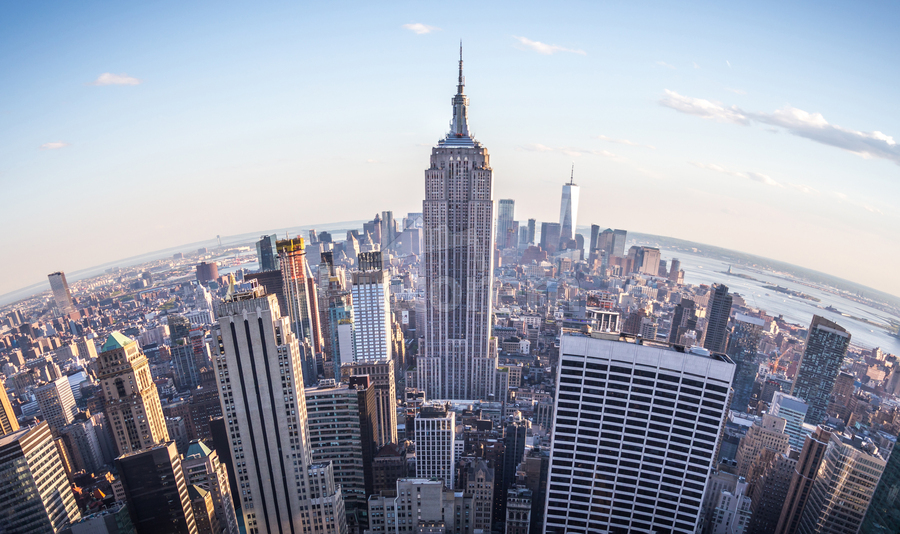This aerial photograph offers a breathtaking view of a bustling city skyline, likely New York City, given the recognizable elements and architectural features. Captured at a slight angle, the rectangular image is dominated by skyscrapers of varying shapes and sizes. The focal point is the tallest building in the center, which resembles the iconic Empire State Building. To the right, a shimmering body of water, possibly the East River, stretches alongside the urban expanse, with bridges such as the Brooklyn and Manhattan Bridges faintly visible, connecting different parts of the city. Pockets of green space, hinting at parks, punctuate the man-made landscape, adding a touch of nature to the concrete jungle. The sky transitions from light blue to a hazy pink near the horizon, enhancing the serene yet dynamic atmosphere. This photorealistic representation, adorned with a semi-transparent white watermark featuring a mountain graphic, captures the city's remarkable human achievement in urban development, akin to marvels like the pyramids, and evokes thoughts of ancient civilizations and lost cultures.